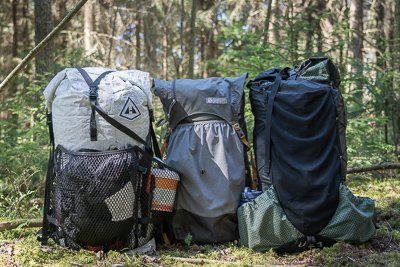The photograph captures three large hiking backpacks, aligned side-by-side, set on a forest floor that is mossy and scattered with dirt and grass. Towering behind them is a thick forest with dense green bushes and an array of brown tree trunks, giving the scene a rich, natural ambiance. 

The backpack on the left is predominantly light gray, featuring a distinctive patch on the top right corner. The bottom portion is made of gray or charcoal-colored mesh containing items, including a prominent orange-and-white drinking cup.

The middle backpack, the smallest of the trio, is darker gray on top with a lighter gray, pouch-like area at the bottom. It has a closed gray flap on top and noticeable straps.

The backpack on the right is the largest, with a dark charcoal color and two large olive green pouches on either side. Each of these high-quality, durable backpacks is designed for serious hiking or camping trips, emphasizing both functionality and rugged use. Despite the detailed gear, there are no people or other objects in the scene—just the serene backdrop of the untamed forest and the trio of backpacks, ready for adventure.